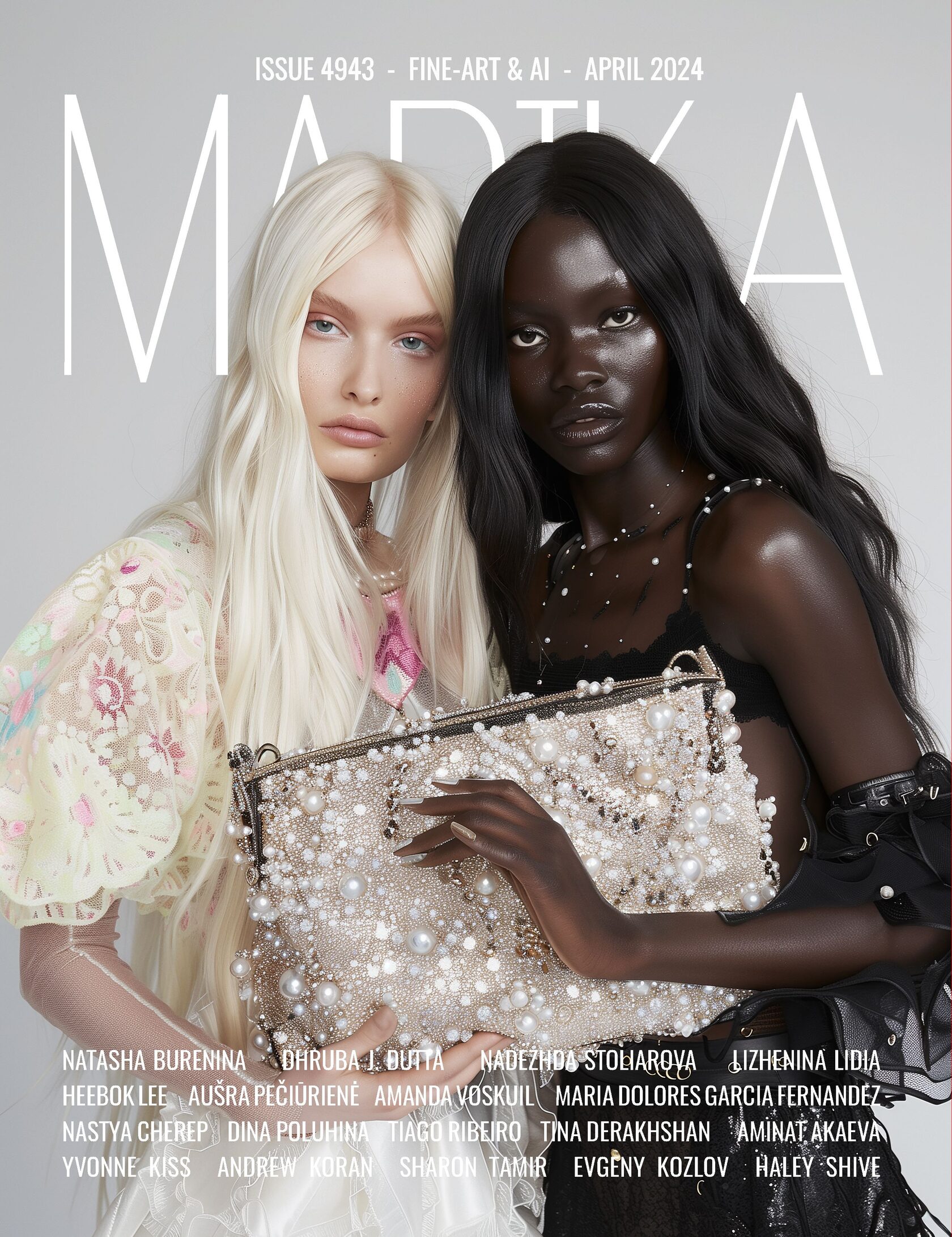This is a vertically aligned rectangular picture resembling a magazine cover, with the title partially obscured by two central figures. The magazine's details, "Issue 4943, Fine Art and AI, April 2024," are clear above the models. The title seems to read "MADTKA," although their heads obscure part of it. The central figures are two women with serious expressions, meeting the viewer's gaze. 

On the left is a fair-skinned woman with blunt, platinum blonde hair parted in the middle, mesmerizing blue eyes, and a lacey white floral dress. To her right stands a dark-skinned woman with glistening skin, dark brown or black hair also parted in the middle, and brown eyes. She dons a scanty black outfit adorned with lace, decorations, and possibly black leather. Both models hold a rectangular bag encrusted with what appears to be diamonds or pearls. Below them, the bottom of the cover lists several names in white text, contributing further to the magazine's detailed presentation. The models’ flawless appearances suggest a highly stylized, potentially AI-enhanced image.